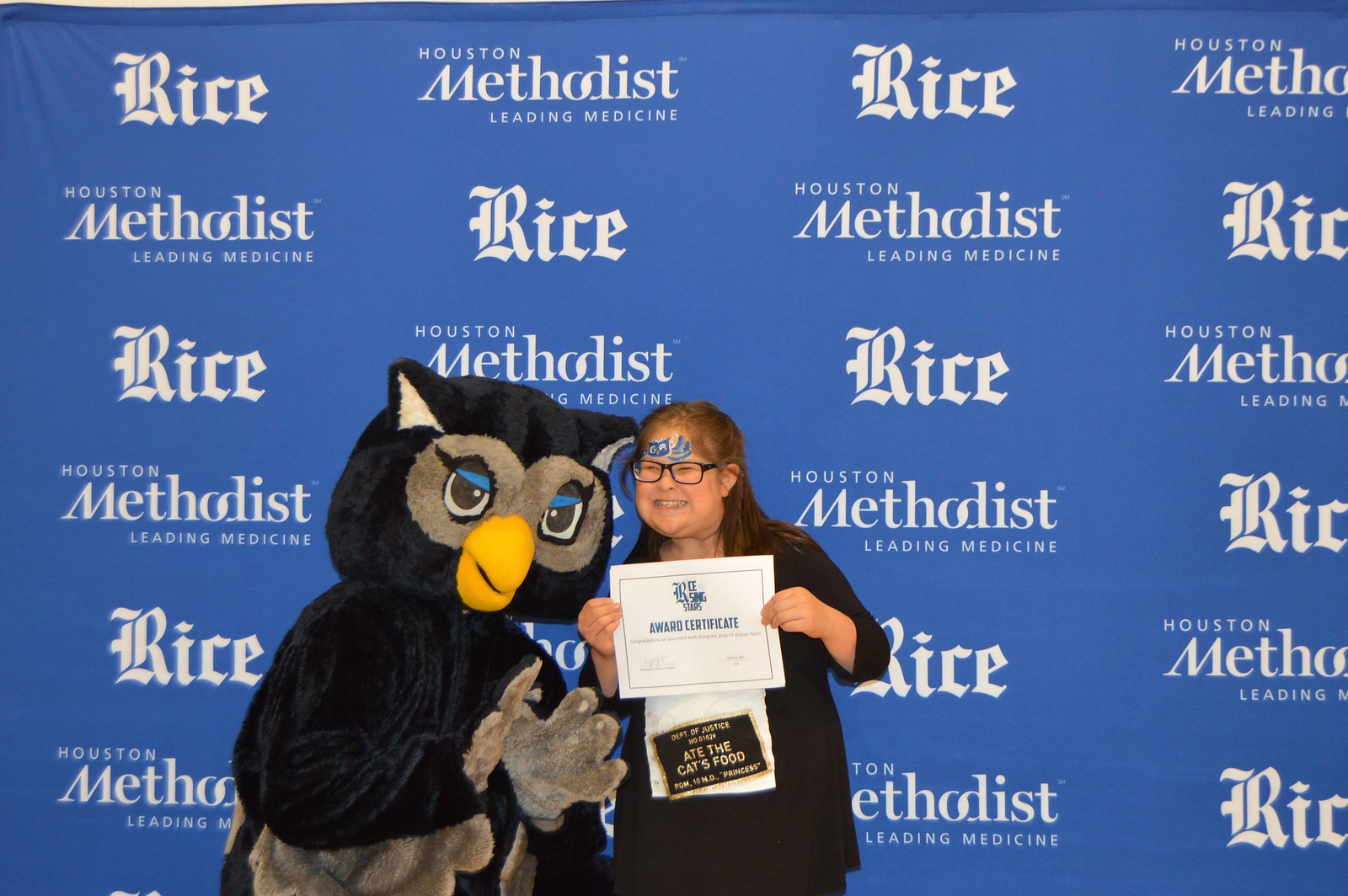In the photograph, a young girl is standing on the right side, proudly holding a certificate in front of her chest. The girl has long dark hair, wears black glasses, and has blue face paint or stickers on her forehead, complementing her cheerful smile. She is dressed in a black jacket, a white shirt with a black rectangle that reads "ate the cat's food, 10 month princess," and black pants. Standing to her left is a mascot resembling the Rice University owl, characterized by a yellow beak, blue and black eyes, and a black and gray feathered body with black and white ears. Both are posing in front of a large blue board with white writing, displaying sponsors such as Rice University and Houston Methodist Leading Medicine.